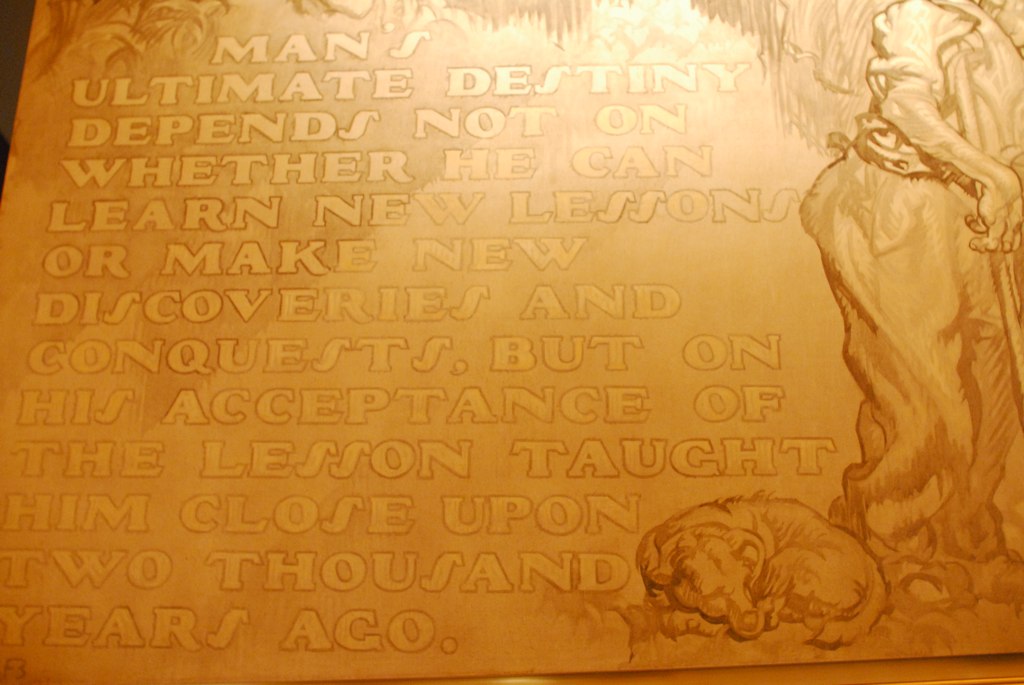The photograph captures a detailed, large carved stone motif on a wall. The stone, predominantly yellowish-gold with a shiny aesthetic, features a relief of a woman dressed in a vintage or Greek style. The woman is positioned on the right side of the image, standing in front of the stone. At her feet, a dog is curled up, appearing to rest peacefully. The stone relief is intricately carved, making the fine details difficult to discern under the heavy lighting.

To the left of the woman, engraved text is visible, although challenging to read due to the lighting and the relief carving. The inscription reads: "Man's ultimate destiny depends not on whether he can learn new lessons or make new discoveries and conquests, but on his acceptance of the lesson taught him close upon 2,000 years ago." This evocative quotation, along with the serene scene of the woman and the dog, creates a reflective and timeless artwork. The colors vary from dark brown lettering to a lighter brown and gold-hued stone, enhancing its historical and artistic ambiance.